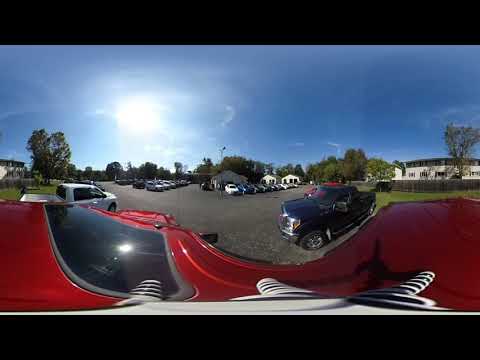The image captures a bustling parking lot scene on a bright, sunny day, framed by thick black borders at the top and bottom. In the foreground, a red vehicle dominates the scene, partially cropped but revealing a black glass window on the left and a white section on the bottom with an indented curve in the middle. Just in front of this red vehicle to the right, there's a dark-colored pickup truck, notably positioned with its front end facing downward to the left. On the left side, closer to the red vehicle, a white dual cab pickup truck is parked with its front end to the right.

In the middle ground, there are rows of parked vehicles, stretching across the image from the left to the right. Specifically, a large black truck with a prominent grill and tire is directly ahead of the red vehicle, while assorted cars fill the spaces beyond. In the far-left center, there's a building that could be an apartment complex, and in the very center of the background, more buildings are visible, perhaps residential. To the right-center of the image stands a large, elongated structure that could also be an apartment building.

The sky above is a clear blue with wispy clouds, suggesting a sunny, likely Sunday afternoon filled with churchgoers. The trees dotting the area add to the pleasant and vibrant atmosphere.